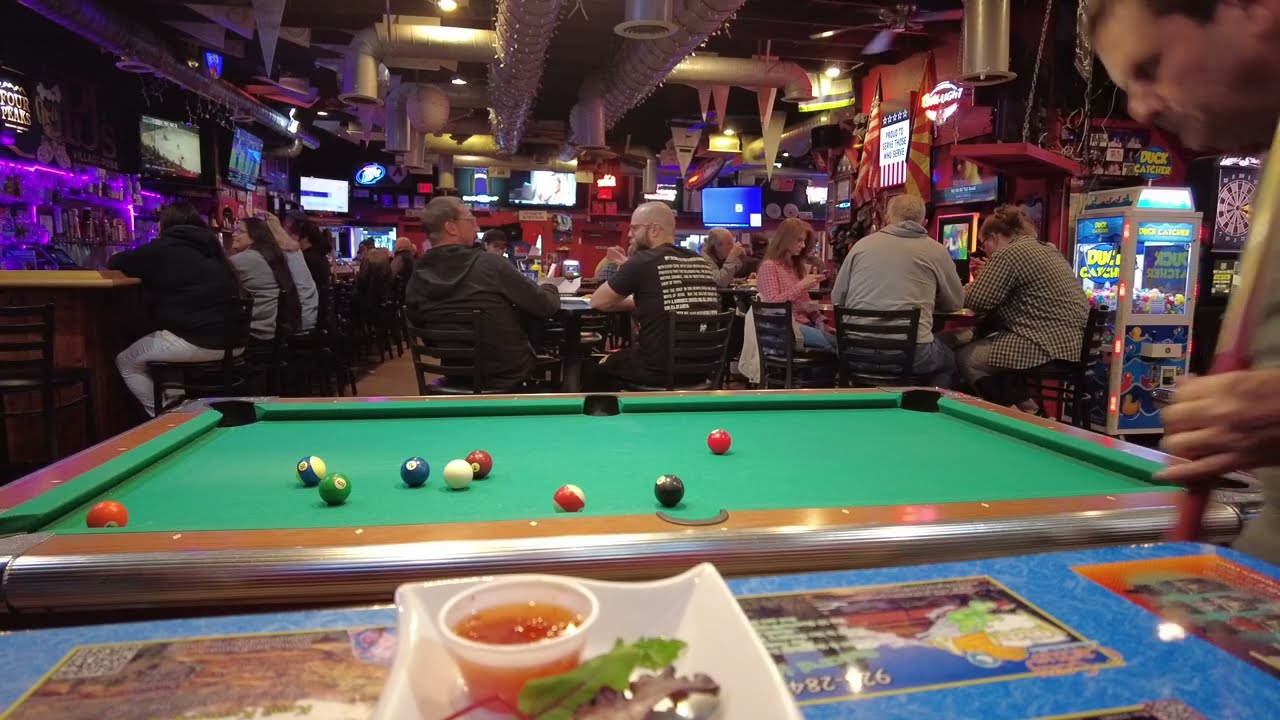This interior photograph captures a lively bar scene with a mix of recreational and social activities. In the immediate foreground, there's a blue tabletop adorned with stickers, holding a white rectangular plate containing a sauce cup and what appears to be a small salad. Just beyond this table, a wooden-framed billiard table with green felt is visible, scattered with billiard balls mid-game. To the right of the pool table, a man with a bearded, blurred face is holding a pool cue in his left hand. The middle section of the image showcases several patrons seated at tables, engaged in conversations and enjoying drinks. To the left of this group is the main bar area, where additional patrons are seated. Notably, a man with short cropped brown hair and another man with long shaggy blonde hair are visible. To their right, a smaller group comprising two men and one woman are seen chatting and drinking beers. On the right-hand side of the image, near a dartboard, there is an arcade or gaming machine. The far background features more seating, with multiple televisions mounted along the walls, although their content is unclear. Overhead lights illuminate the lively atmosphere of the bar.